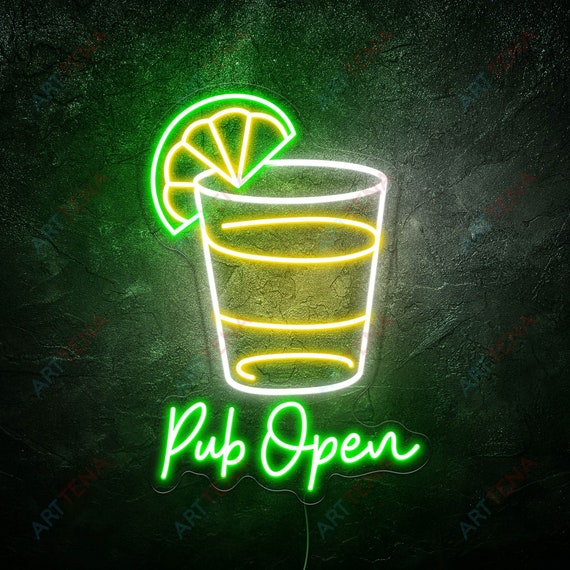In this detailed image, we see a vibrant neon sign against a dark, possibly textured black background. The illuminated centerpiece features a white neon outline of a drinking glass, which contains curved yellow neon bands suggesting a beverage. At the top left of the glass, a vivid slice of lime, depicted with green and yellow neon lights, rests on the rim. Beneath the glass, the words "Pub Open" are elegantly written in cursive using green neon lights. The entire neon display casts a gentle glow, gradually fading into the dark background. This striking and colorful neon sign is characteristic of those typically found in bar windows or tailored man caves, adding a lively and inviting atmosphere. A small, unobtrusive cord dangles from the sign, completing the setup.